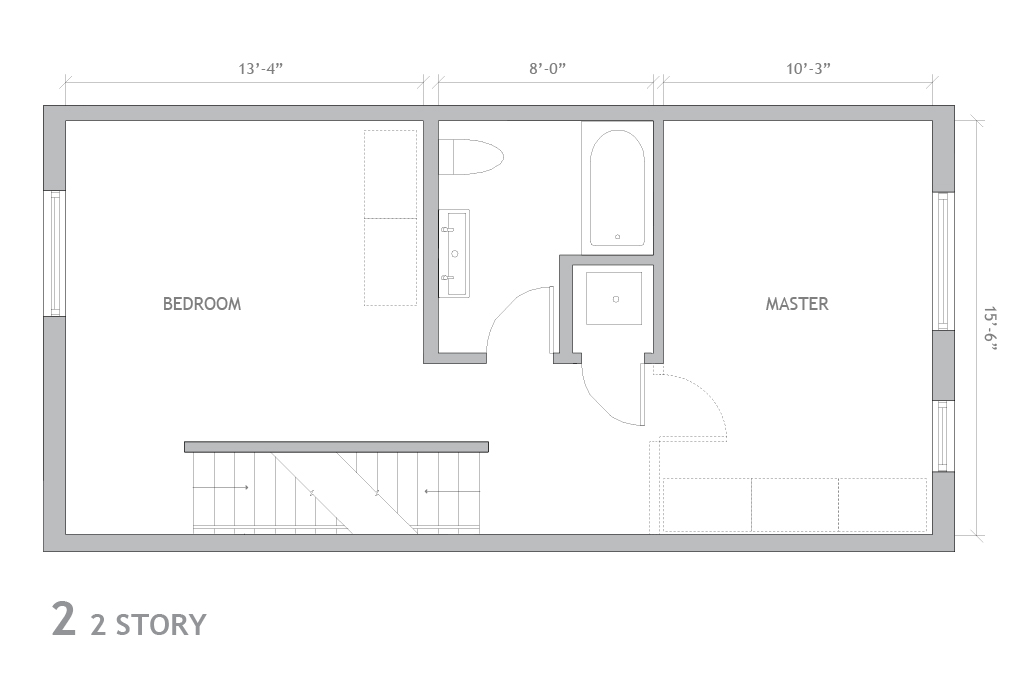This image depicts a detailed floor plan for a two-story house, rendered in shades of white and gray. The blueprint is oriented horizontally, stretching left to right in a rectangular shape. 

On the left side of the blueprint, there is a large square area marked as a bedroom, measuring 13 feet 4 inches in length. This room appears to have an opening on the left, likely a window. Situated at the bottom of the bedroom is a staircase, suggesting access to another level.

Adjacent to the bedroom is a bathroom, with dimensions of 8 feet 0 inches. The bathroom layout includes a sink, a toilet, a bathtub, and a closet, clearly delineating the necessary amenities.

To the right of the bathroom, there lies the master bedroom. The master bedroom spans 10 feet 3 inches at the top and extends 15 feet 6 inches to the right. These measurements define a spacious area, likely designed for comfort and ease of movement.